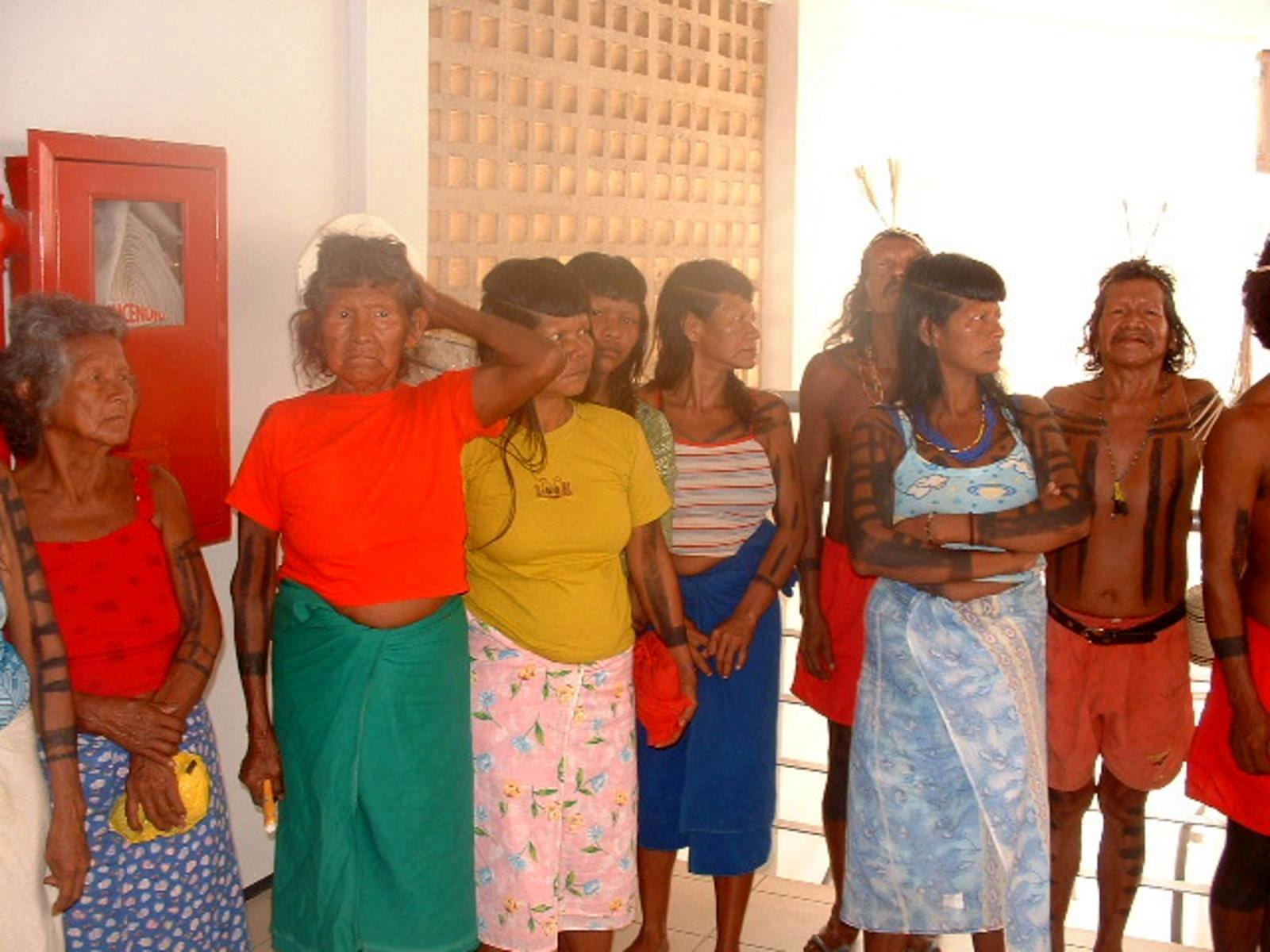The photograph captures a diverse group of about nine or ten individuals, consisting predominantly of women with two to three men, who appear to be Indigenous or Native American. They are gathered outside on a bright, sunny patio adorned with a beige, textured wall of repeating squares, and a noticeable fire extinguisher mounted nearby. The men are shirtless, their bodies decorated with traditional paint and feathers, while the women wear a mix of skirts and colorful modern clothing, also featuring arm paint or tattoos. Most individuals are looking off to the side, giving an impression of being distracted or engaged in something beyond the frame, with only a couple of them facing the camera. This gathering, marked by cultural attire and body art, stands against the backdrop of an eclectic setting, which includes a fire hose encased in a red box, concrete structures, and large windows letting in ample sunlight. The group's expressions range from neutral to slightly displeased, creating a scene rich with cultural significance set in a modern context.